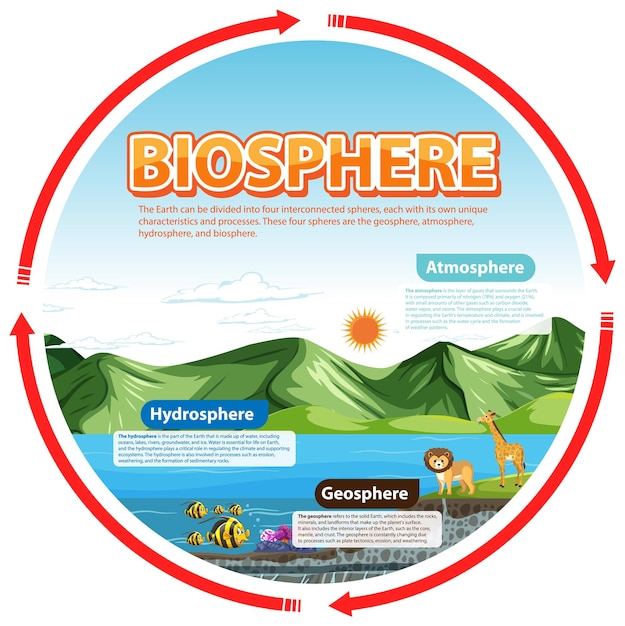The image is a detailed, circular diagram titled "Biosphere," illustrating how the Earth can be divided into four interconnected spheres: the geosphere, atmosphere, hydrosphere, and biosphere. The diagram features a blue sky with white clouds, a sun situated above green hills, and blue water. Red arrows encircle the entire image, symbolizing the interconnected nature of these spheres.

On the right side, the word "Atmosphere" is written in white letters on a blue background. The left side features "Hydrosphere" in white letters on a darker blue highlight, placed over the blue water. At the bottom, "Geosphere" in white letters is overlaid on brown terrain. The diagram depicts fish swimming in the water, and on green land, there are animals such as a lion and a giraffe. Overall, this illustration emphasizes the interdependence of Earth's spheres, combining visual elements and textual descriptions to convey their distinctive characteristics and processes.